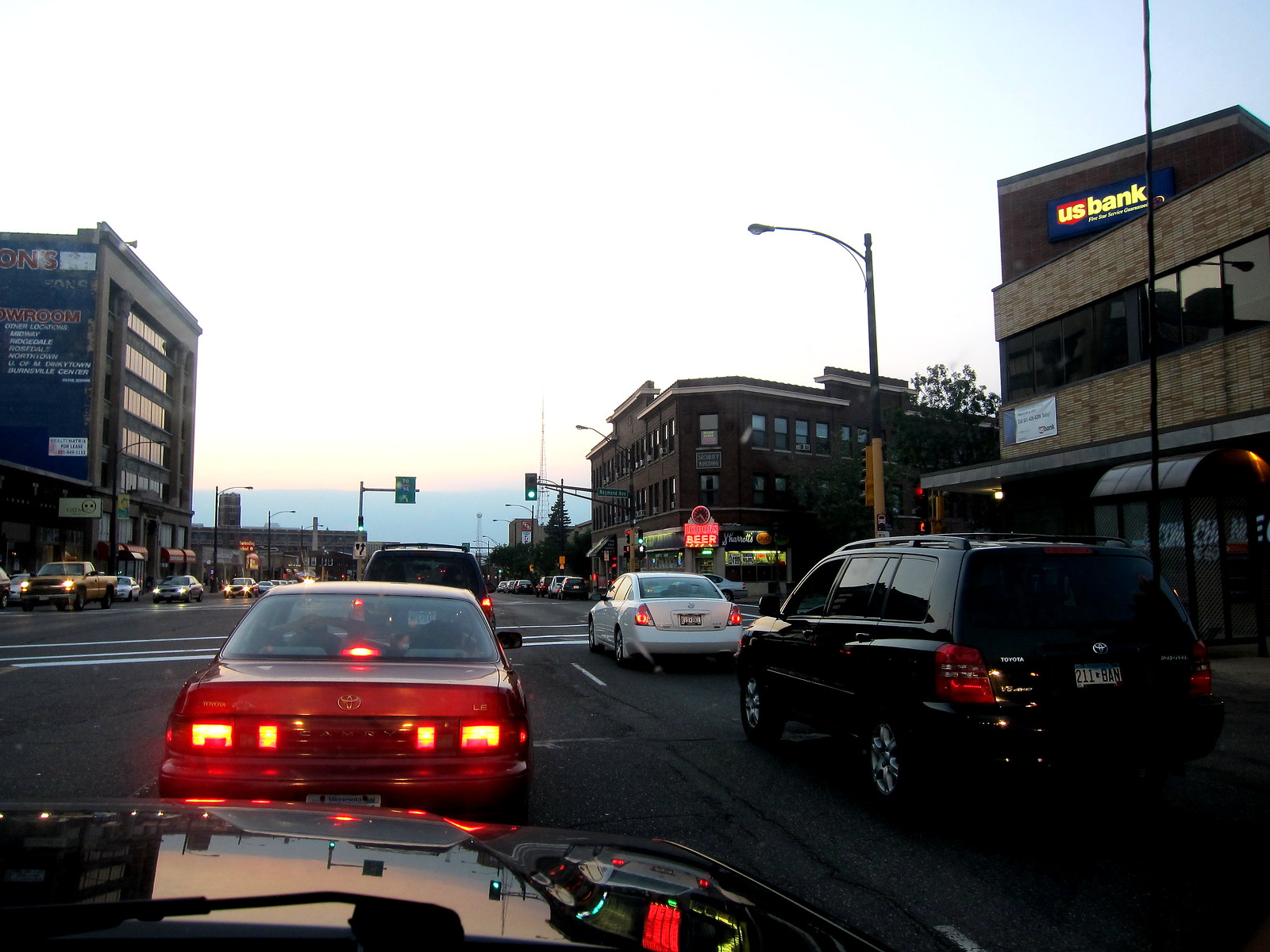In this dash cam photograph, taken from the perspective of a black car at an urban intersection, the viewer can see the reflection of a sky transitioning between night and day, characterized by a washed-out whitish-blue hue common during sunrise or sunset. The vehicle lights are all turned on, suggesting dim lighting conditions. The intersection is set within a bustling cityscape, flanked by multi-story buildings on three visible sides. Directly ahead, a red Toyota waits at the crossroads, with a black SUV to its right and a white sedan positioned in front of the SUV. Ahead of the Toyota, another dark 4x4 vehicle is poised to move as the traffic lights have just turned green. Among the buildings, a prominent sign reads "US Bank," and a lit-up cafe or coffee shop sign is visible diagonally across the intersection, contributing to the vibrant yet tranquil ambiance of the scene.